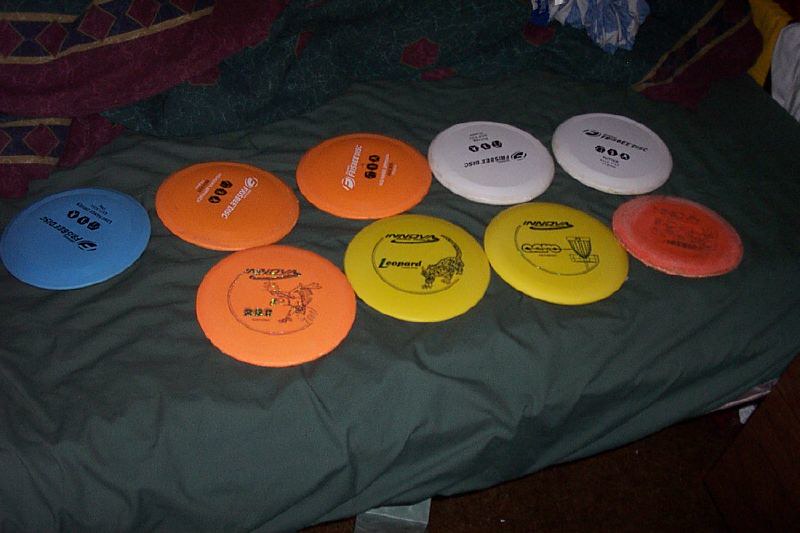The photograph showcases nine disc golf frisbees neatly arranged on a blue sheet, which appears to be spread either on a bed, couch, or table. The setting is in a room with a dark red or brown floor, featuring a red blanket and various, hard-to-discern pillows in the background. The frisbees come in different colors and are laid out in a loose pattern: a solitary blue frisbee on the left, followed by pairs of orange, orange and yellow, white and yellow, and finally white and red frisbees. Each frisbee is adorned with text and images, including distinct designs such as an eagle, a leopard, and a frisbee golf goal cage. Although the exact details of the text and imagery are challenging to decipher, the markings likely represent brand names and logos related to disc golf.